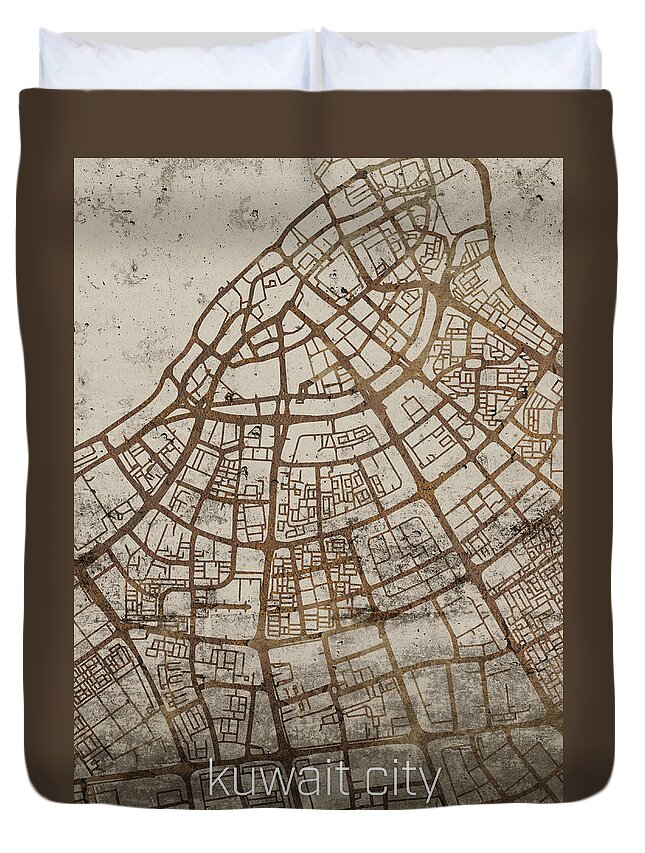The image depicts a detailed map of Kuwait City, presented in a format that might be a form of textile or a textured paper with a dark brown border. The map itself is primarily in an off-white or very light brown color, surrounded by the dark brown gradient expanding from dark to medium to light brown tones. The geographic area of Kuwait City is shaped somewhat like a mountain or an inverted V, fanning out with streets and intersecting roads.

The streets form a grid that isn't perfectly rectangular, comprising various diagonal and semicircular bands. Approximately five significant roads radiate and converge diagonally toward the top-middle part of the map. In between these roads, additional streets and buildings are illustrated in various shades of brown, with lighter brown lines outlining numerous buildings. At the bottom of the map, the text "Kuwait City" is clearly visible in white. 

The background suggests the map is laid over a surface that has visible white bricks at the top, hinting that it might be mounted on or part of a flyer. Despite the urban layout, no additional labels or texts are present on the map except for the city's name, making it a purely visual guide to the streets and structures of Kuwait City.